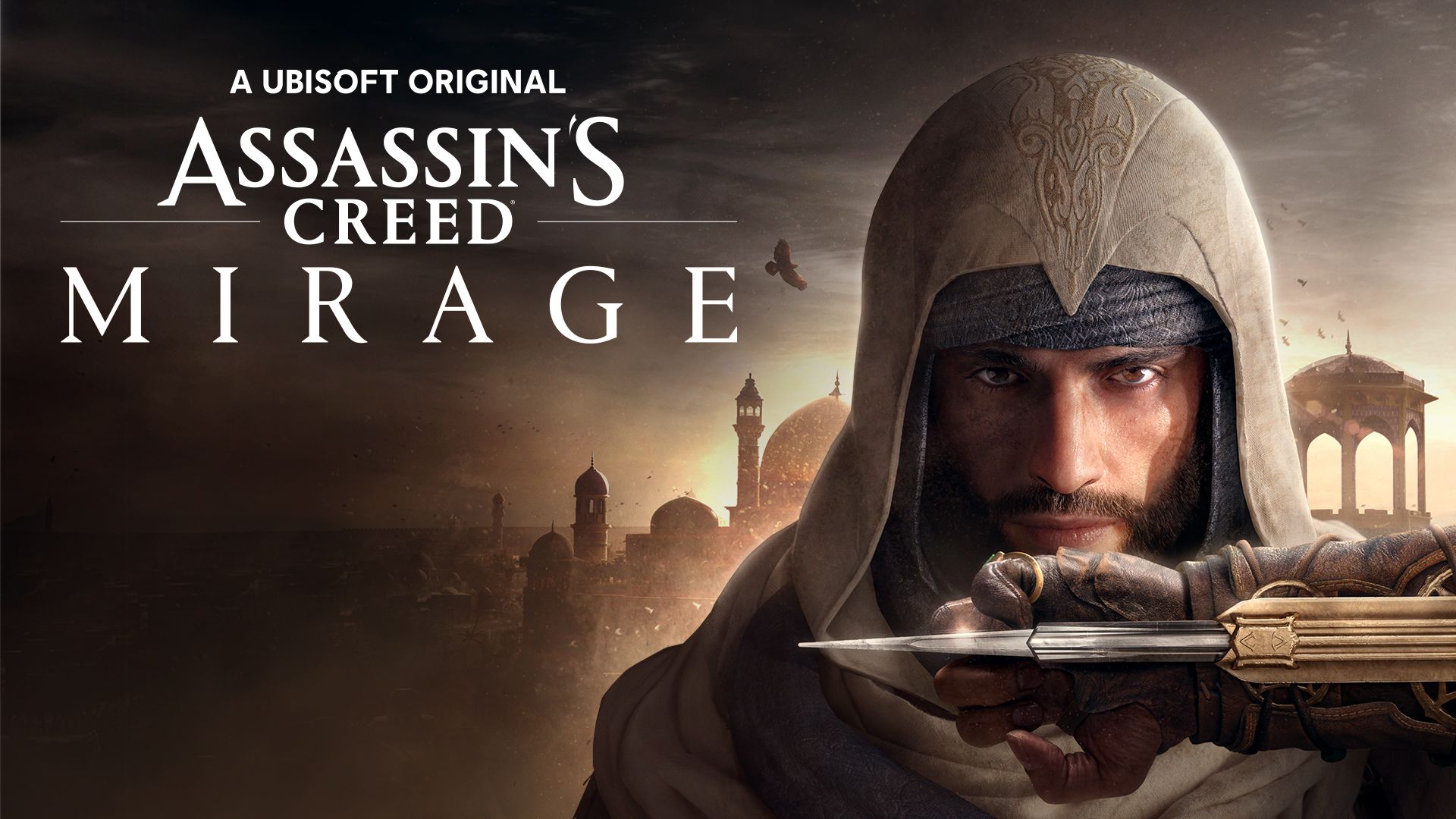This image is an advertisement for the Ubisoft video game, Assassin's Creed Mirage. In the top left corner, white text reads "A Ubisoft Original" with "Assassin's Creed" underneath, followed by "Mirage." The main focus is a close-up of a medieval man with a serious expression, staring directly into the camera. He is wearing a brownish hoodie with intricate designs carved into it, layered over another grayish hoodie. The man has a dark mustache and beard, along with a helmet and a knit or woven hat beneath it. His left hand, covered in what appears to be a heavy armored or leather glove, is raised near his face, palm towards the camera, revealing a long silver dagger extending from a golden wrist attachment. In the background, there are vague outlines of Middle Eastern architecture, including buildings and possibly a gazebo, with colors consisting of blue, brown, white, grey, navy, silver, yellow, and hints of red.